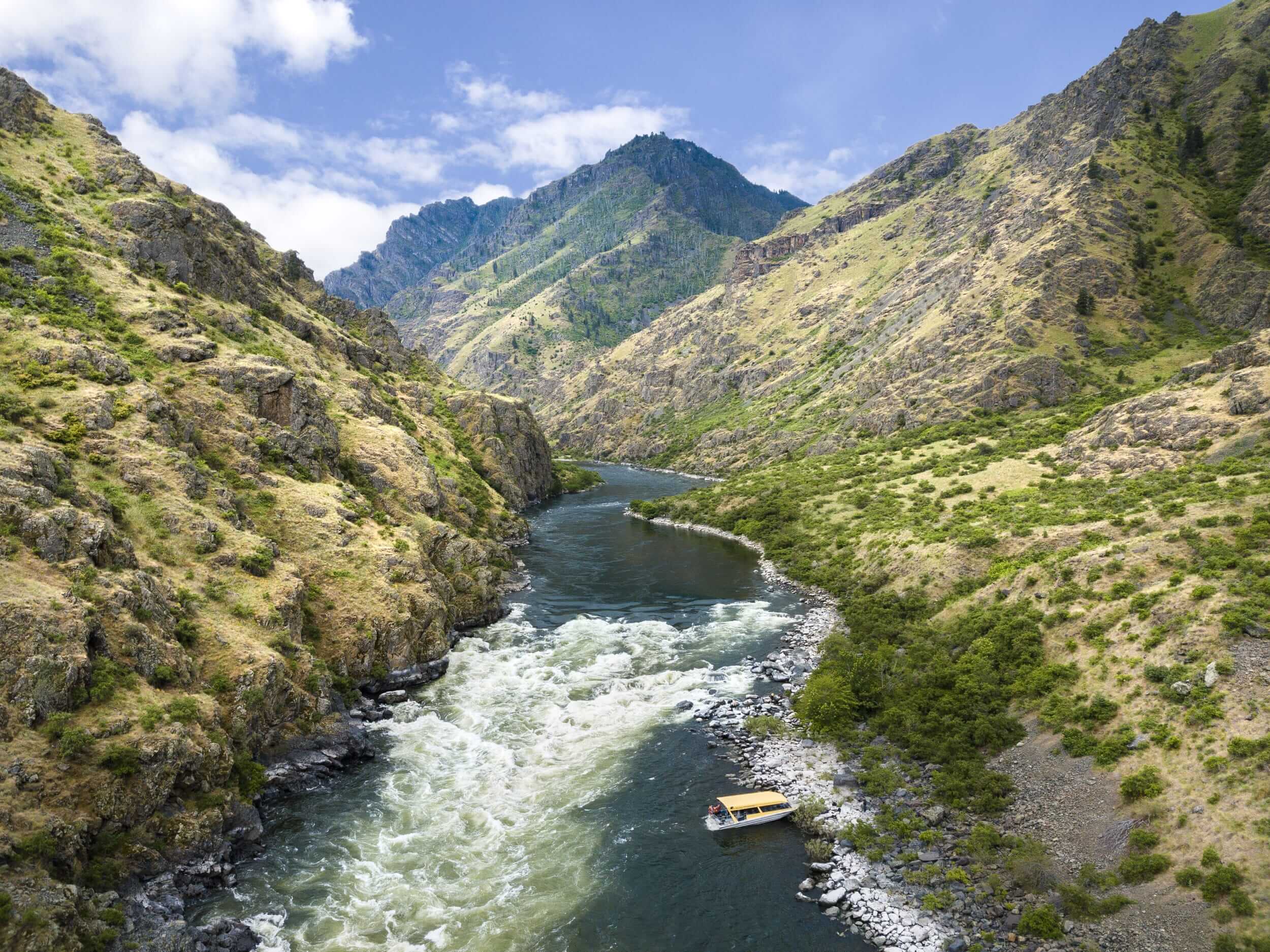The image captures a stunning mountainous landscape with several large, rocky mountains interconnected at their bases. The mountains feature a tapestry of grey rocks, green shrubbery, and patches of tan grass, indicative of a late summer or early autumn setting. At the heart of this scenic vista flows a winding river, its water a greenish-brown hue, gushing and choppy, with visible foam from the waves. Along the riverbank, particularly to the right, there is a vibrant array of green vegetation and plants, interspersed with rocks. To the left, similar rocky formations and greenery rise to meet the mountains.

At the bottom of this river, nestled within a basin, sits a small boat. The boat features an orange-beige canopy and a silvery lower deck, with a man seated at the back, appearing stationary on white rocks adjacent to the river's edge. In the background, towering mountains continue to cradle the river, their rugged surfaces marked by small cracks and formations. The sky overhead is a clear blue, adorned with wispy clouds drifting in from the left, bathing the entire scene in sunlight and enhancing its natural beauty.